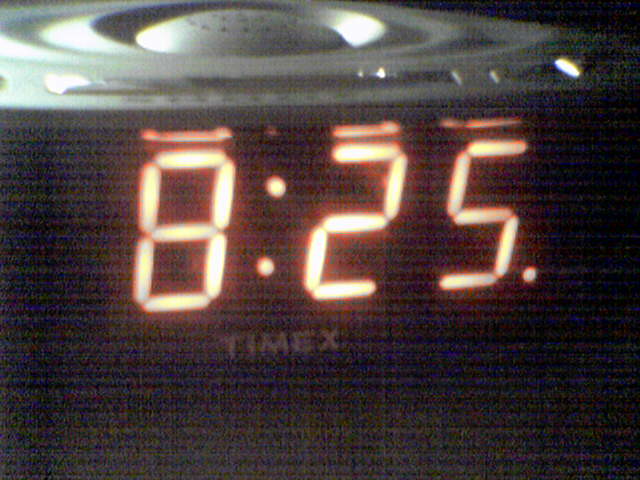A high-quality, dimly lit photograph features a Timex alarm clock prominently. The clock face displays the time "8:25" in bright red LED digits. The brand name "Timex" is clearly visible in white text beneath the time display. The image also captures a speaker positioned on the top of the clock, hinting at additional functionalities.